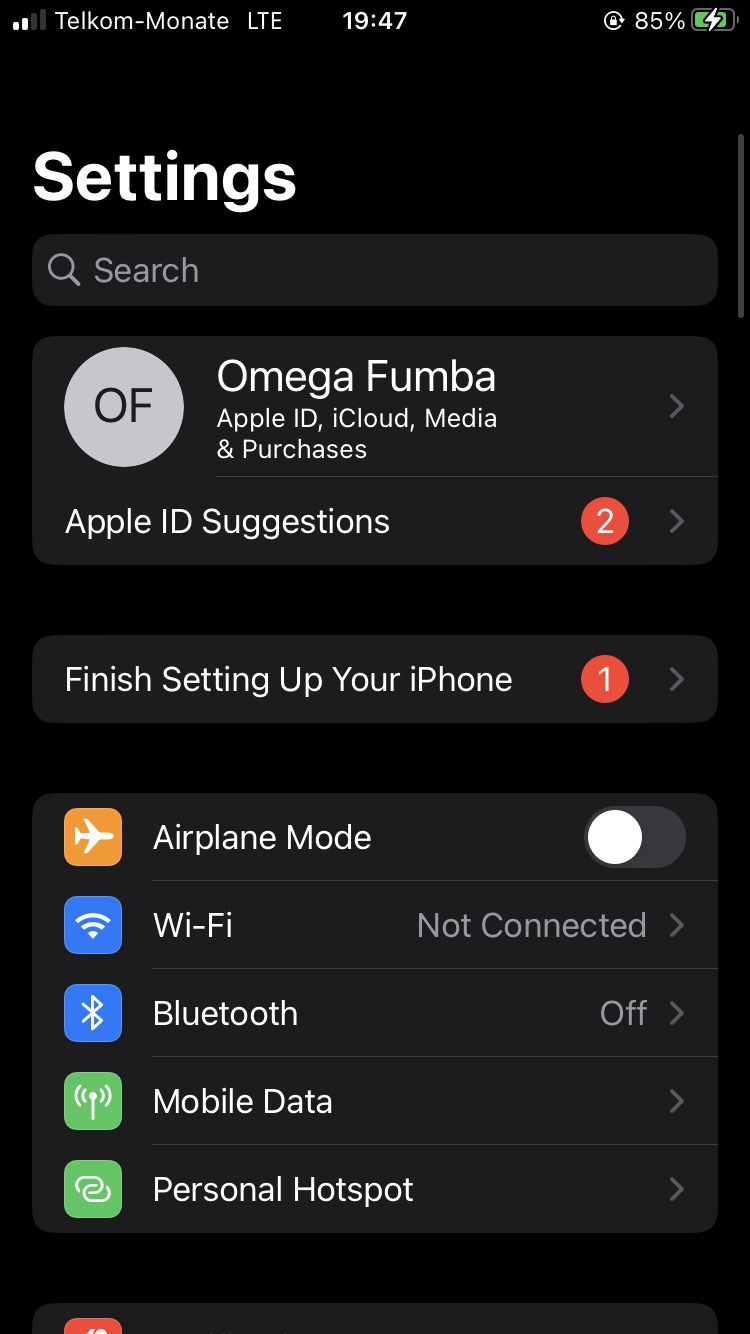An image depicts a black smartphone against a completely black background. The phone's status bar at the top displays various essential indicators: the signal bars show connection strength and the carrier name "Telecom Monet LTE," the current time is "19:47:47," and the battery level is at "85%" depicted with a green battery icon.

Beneath the status bar, the first word displayed in bold white text is "Settings." Below it lies a dark gray search box with a magnifying glass icon for searching. Following this, different settings options are listed. 

The first option reads "Omega Fumba, Apple ID, iCloud, Media, and Purchases," accompanied by a gray circular icon with the initials "OF" to its left and an arrow on the right for further navigation.

Next, "Apple ID Suggestions" is positioned, with a red circular notification badge displaying the number "2" and an arrow to its right. Below, it states "Finish Setting Up Your iPhone," marked with a red circular notification badge with the number "1," and an arrow accompanies it on the right.

Further down, the "Airplane Mode" setting is apparent with an orange icon featuring a white airplane on the left and a switch to toggle on and off on the right.

Subsequent settings are "Wi-Fi Not Connected," denoted by a blue Wi-Fi icon, and "Bluetooth," identified by a respective icon, which is currently off. The "Mobile Data" option is in green with its corresponding icon, and "Personal Hotspot" follows, each equipped with navigation arrows.

The view does not capture the very bottom of the phone, leaving some details out of sight.